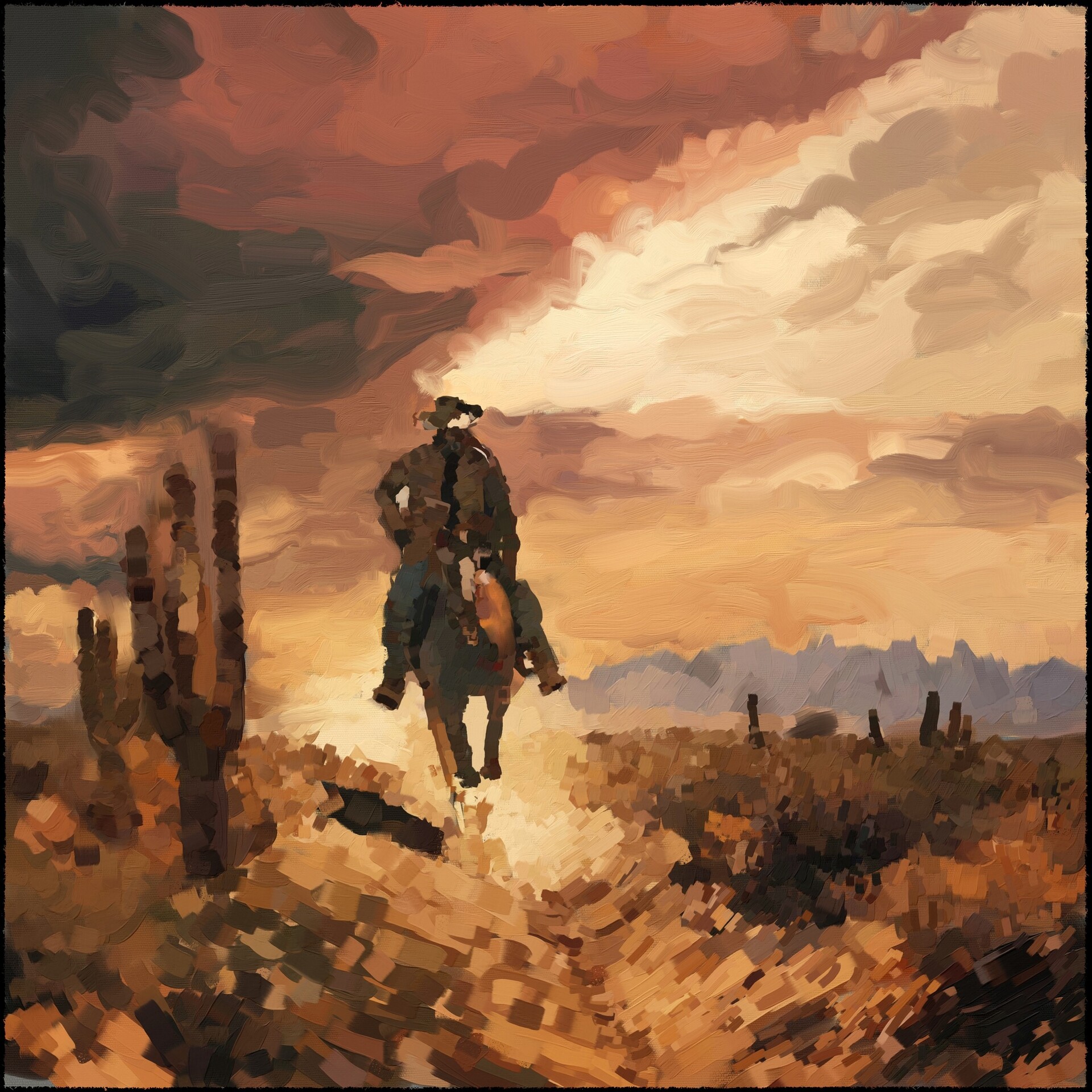This vibrant, mosaic-inspired painting captures a dramatic desert southwestern scene dominated by varying shades of brown with occasional hints of purple. At the heart of the artwork is a cowboy riding a horse, both figures moving forward with their backs turned towards the viewer. The cowboy is dressed in a brown jacket, blue jeans, brown boots, and a distinctive cowboy hat. The composition includes two cacti on the left side, while the right side features distant mountains and rocks under a sky transitioning from dark to light hues, accentuated with purplish clouds near the horizon. The mosaic-like patterns of squares and shapes add a unique, artful touch to this detailed depiction of a lone rider in the arid landscape.